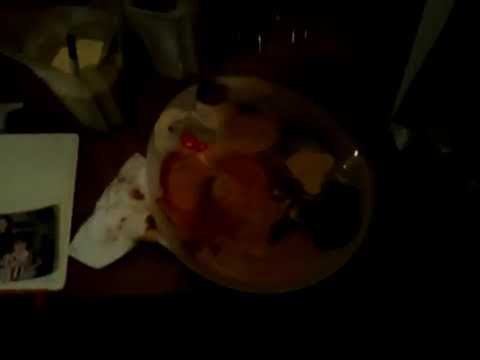The image is a very dark and blurry rectangular photograph, predominantly black in the background, featuring a poorly-lit surface with several objects. In the center, there's a round vessel, likely a plate or bowl, containing a liquid with foam and a distinct red hue on its left portion. The liquid also seems to have objects protruding from it. To the left of this vessel, there is a stained napkin, and further to the left, a white object resembling a coaster or sheet with a possible Polaroid picture near the bottom. Just behind this is a glass containing a lemon and a black straw. The overall photograph appears cluttered and is challenging to see due to the low quality and poor lighting.